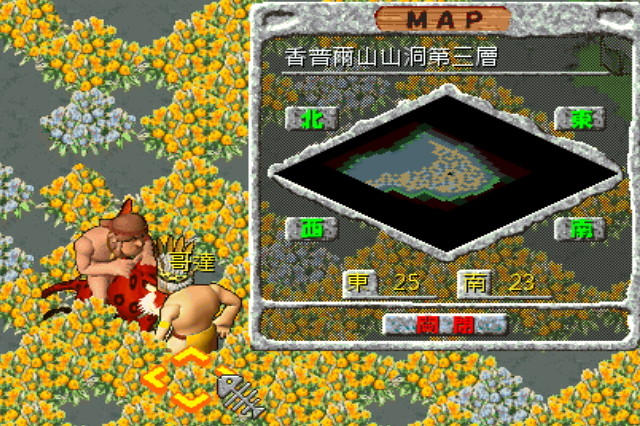This screenshot from a retro-style video game features a vibrant, colorful scene dominated by shades of yellow, brown, and light blue. The background depicts a field filled with what appear to be yellow trees or bushes, contributing to the scene's lively and cartoonish aesthetic. On the left side of the image stand two shirtless, cartoonish characters, presumably of Caucasian descent. The character on the left is shown riding a striking red tiger. Below this rider, there is a yellow box, while a small fish skeleton, which might serve as a cursor, is visible at the bottom of the image.

To the right of the characters, there's an overlaid map box that adds a layer of complexity to the scene. The top of this box is labeled "Map" in black text on a brown background. The map box itself features a border with a white and gray rocky texture, framing a central area with a black background, also encased in the same rocky texture, arranged in a diamond shape. Surrounding the map are numerous smaller boxes filled with long green text. Aside from the word "Map," all other text appears to be in an East Asian script, possibly Chinese or Japanese, indicating that the game might have been developed or set in an East Asian cultural context.